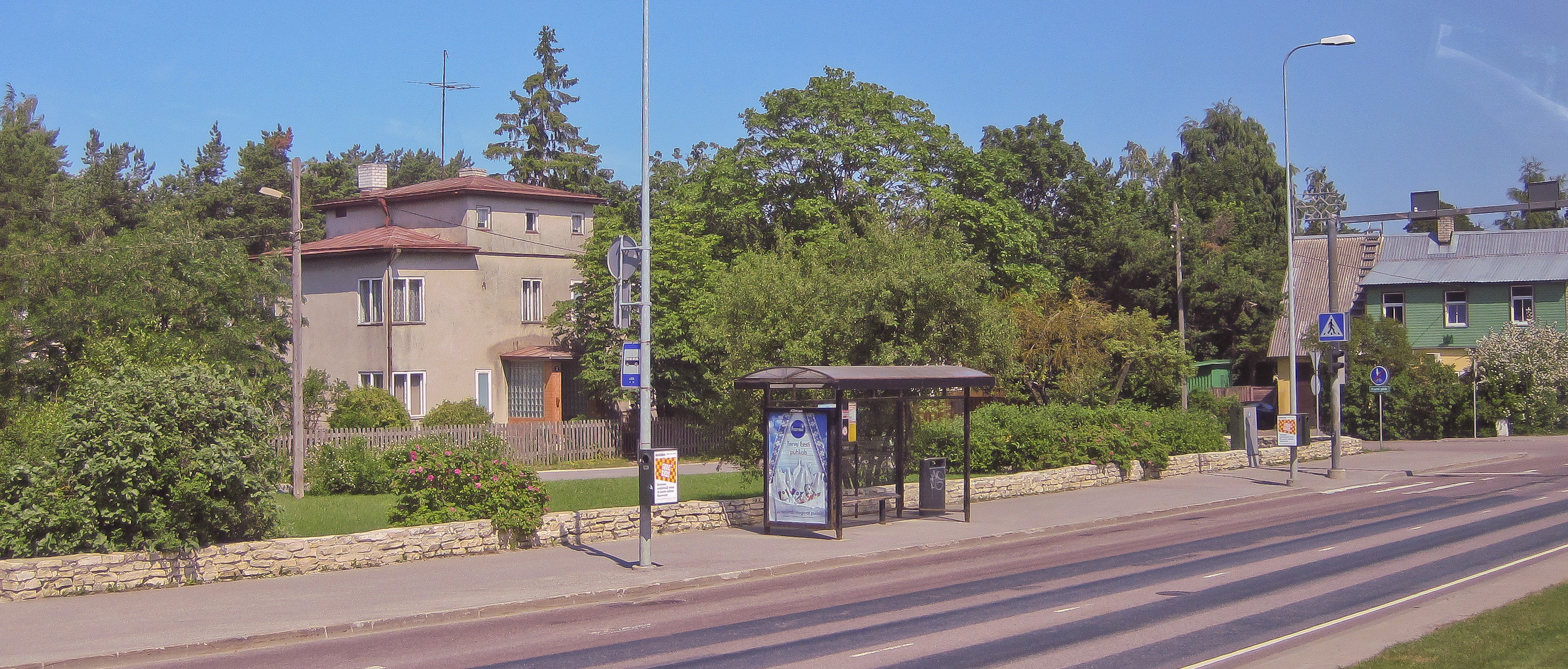The image depicts a quiet suburban street featuring a gray, deserted roadway with noticeable black striping and flanked by sidewalks. Central to the scene is a bus stop with a gray, black metal structure, and a blue billboard advertisement on its left side. Adjacent to the bus stop is a gray trash can. Behind the bus stop, there is a well-maintained lawn adorned with shrubs and a retaining wall made of tan stone. The backdrop showcases a variety of green trees and clear blue skies, enhancing the tranquil atmosphere.

On the left side of the image stands a three-story beige house with a red roof, which appears almost stucco-like in texture. In the foreground, a neatly manicured yard displays a bush with pink flowers. The right side hosts a green building with a sloped, gray, tin roof. Gray street lamps and blue traffic signs punctuate the sidewalks, adding functional elements to this residential tableau.